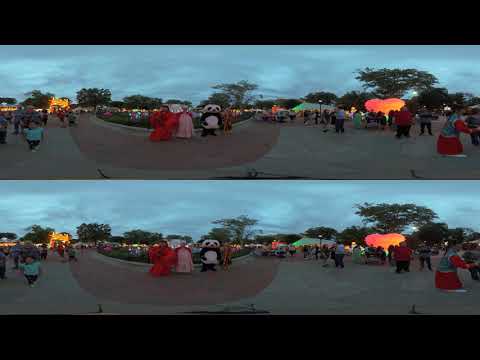The image consists of two identical panoramic pictures, one positioned above the other, depicting an outdoor festival or fiesta. Both images share a fisheye lens perspective, showcasing a vibrant scene with various costumed individuals at the junction of a circular, semi-circular pathway illuminated by brilliant lights beneath the trees. 

In the center of the image stand three prominent figures: one in a striking red dress, another in a white and red dress, and a third dressed as a panda bear. Nearby, to the right, a woman in a blue and red dress can be seen amidst festival-goers walking around what appears to be a stand. Dominating the scene are distinct light features, including an orange light under a tree on the right and a series of lights dotting the background on the left. 

Additionally, a large, fruit-like decoration on the right side of the image is illuminated from within, enhancing the festive atmosphere. The setting also includes a paved path made of two-toned bricks and a backdrop of trees. The sky varies from darker in one image to a lighter blue in the other, suggesting a transition from day to evening under an overcast sky, with grey clouds indicating the approach of night. In the left section of the image, a child wearing a CN t-shirt is visible, accompanied by more people who seem to be enjoying and appreciating the event's scenery.